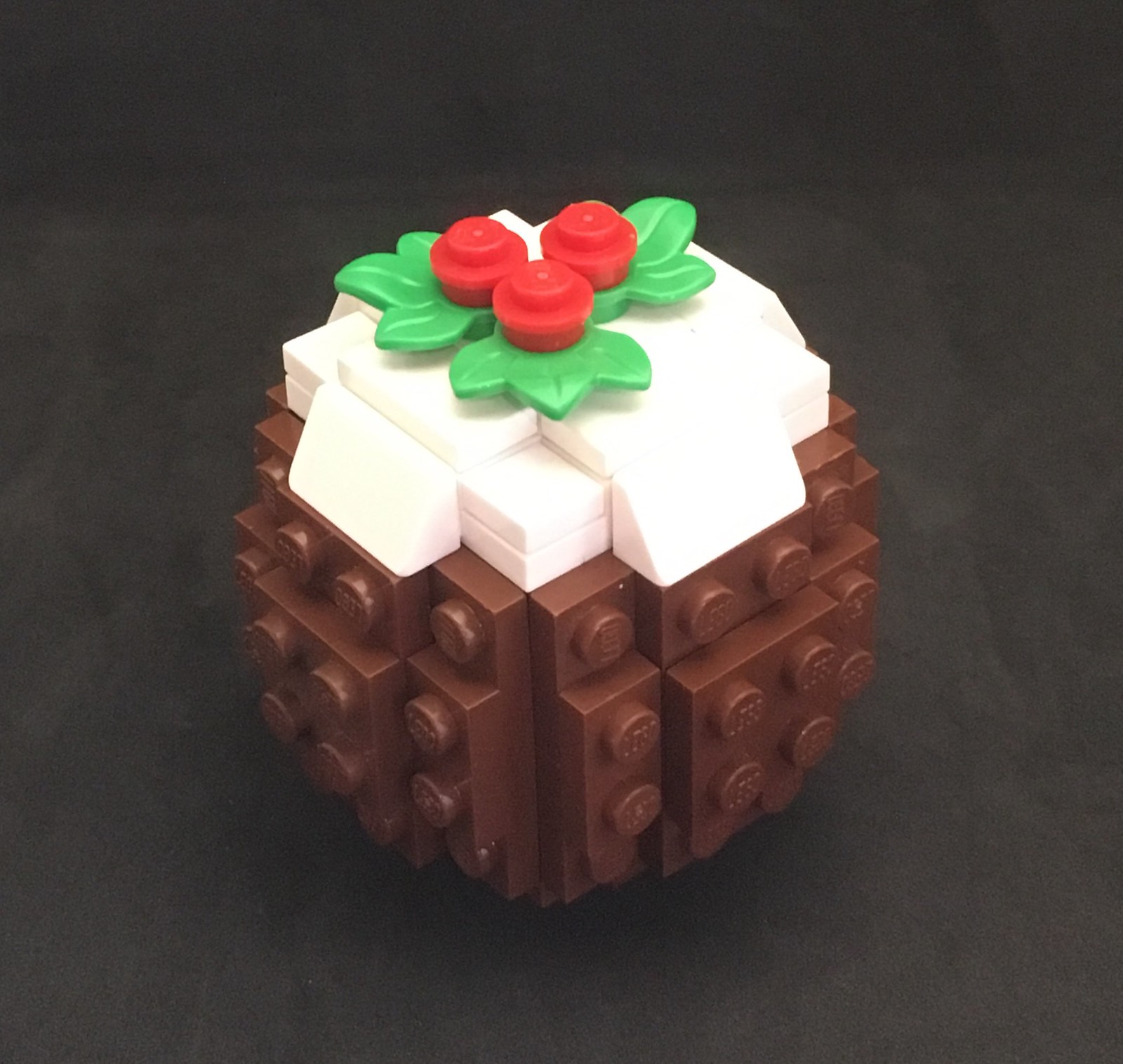This image features an extreme close-up of a small, meticulously crafted Lego sculpture resembling a round chocolate cupcake or bon-bon. The base of the sculpture is constructed from dark brown Legos to mimic chocolate, and the flat top is adorned with white Lego pieces arranged to resemble cream frosting. Crowned with three mint green Lego leaves, the topmost layer includes three small, red Lego pieces, positioned like cherries. The sculpture's compact size suggests it might be only a few inches across, approximately the size of a strawberry or small piece of candy. Set against a stark black background, the detailed Lego creation stands out prominently, showcasing the intricate design and cute appearance.